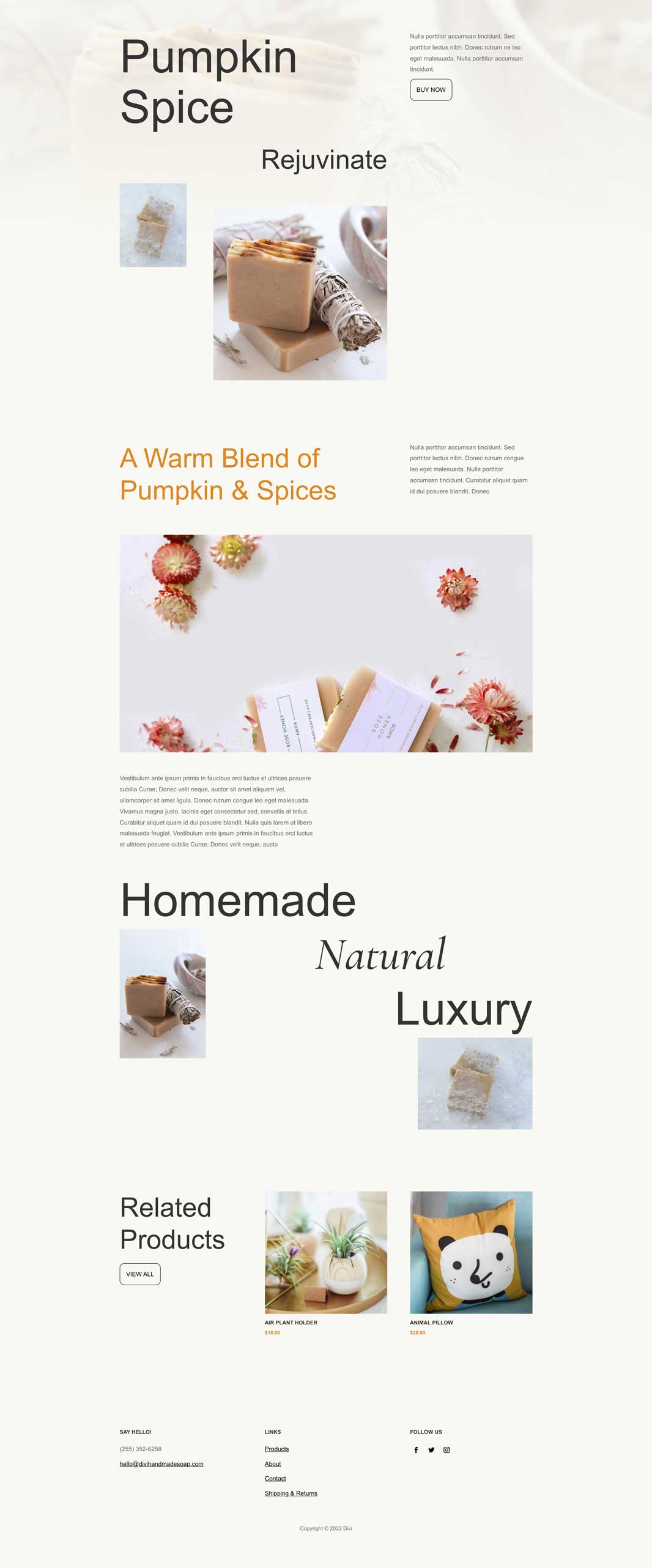The advertisement, displayed on a white background, features "Pumpkin Spice" in the top left corner with "Rejuvenate" positioned just below it. Below this text, a warm, orange-colored caption reads, "A Warm Blend of Pumpkin and Spices," accompanied by images of a pumpkin soap bar next to sage and two varieties of soap bars. Additional text in a foreign language is situated underneath these images. The next section showcases red and white flowers alongside more soap bars, accompanied by similar non-English text. Following this, "Homemade Natural Luxury" is prominently highlighted, with further images of soaps displayed in a repeat pattern. The section titled "Related Products" features pictures of a panda on a pillow, household items such as a serving tray and vases. The bottom part of the page includes social media icons and links to Facebook, Twitter, Instagram, product information, and contact details.